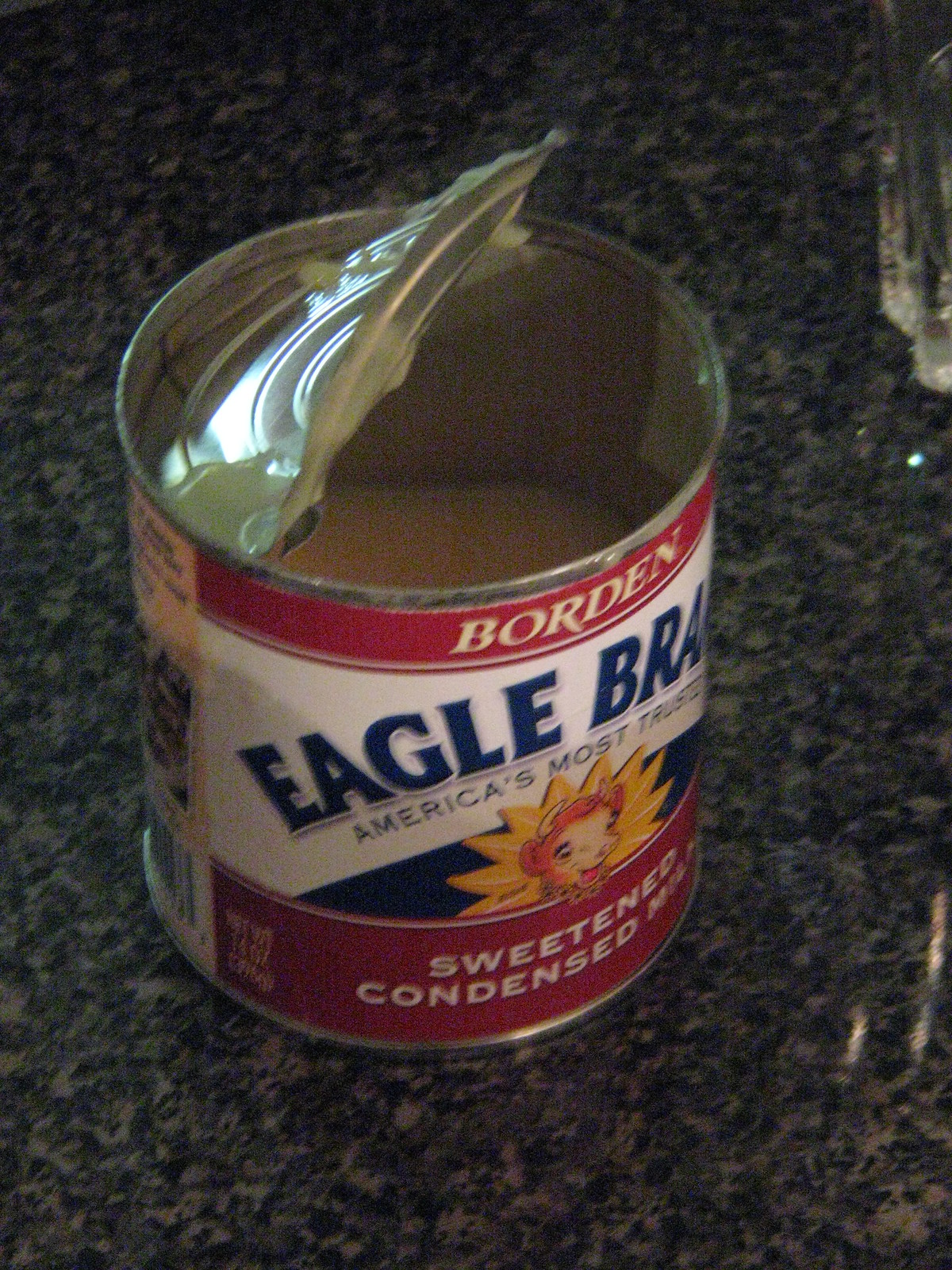In this image, we see an opened can of sweetened condensed milk with a partially used content. The can itself prominently features the brand "Eagle Brand" in large blue letters at the top of a red label. Directly below this, the phrase "America's Most Trusted" is visible, reinforcing the product's reputation. Accompanying these words is an animated, smiling cow, which adds a playful and friendly touch to the packaging. Below the cow, the label clearly states "Sweetened Condensed Milk" in white letters. Toward the top of the can, within the red section, the name "Borden" is printed, likely indicating an association or distribution partnership with Eagle Brand. The can's lid is partially open, revealing that about half of the creamy, sweetened contents have already been used.